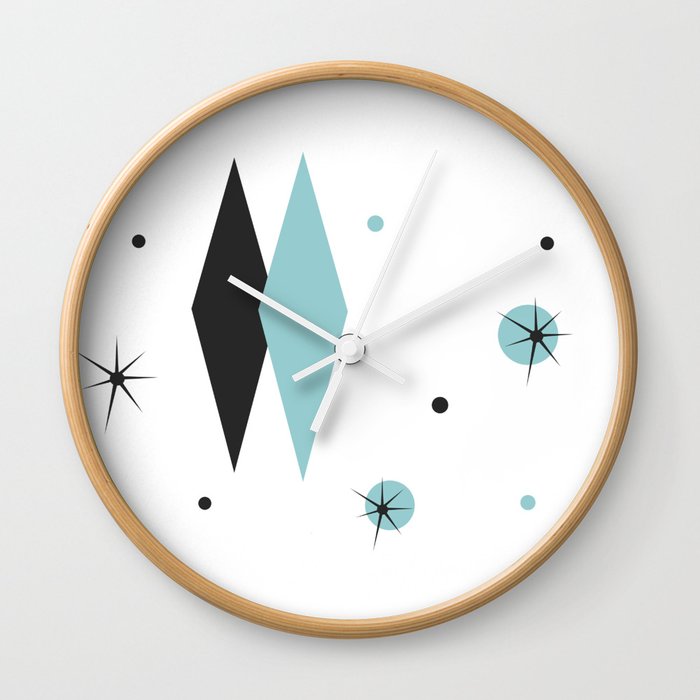The image showcases a decorative and abstract clock mounted on a white wall, framed by a light tan wooden rim. The clock's face, featuring a white background, is devoid of any numbers and instead adorned with a variety of artful patterns. Central to the design are two large, overlapping diamond shapes—one black and the other a pale turquoise. Scattered around these diamonds are multiple black and blue circles along with several black stars. A few of the circles also contain black starburst patterns. The clock has three white hands representing the hour, minute, and second. The overall aesthetic of the clock leans towards a 50s modern style, making it an eye-catching piece of wall art rather than a traditional timekeeping device.